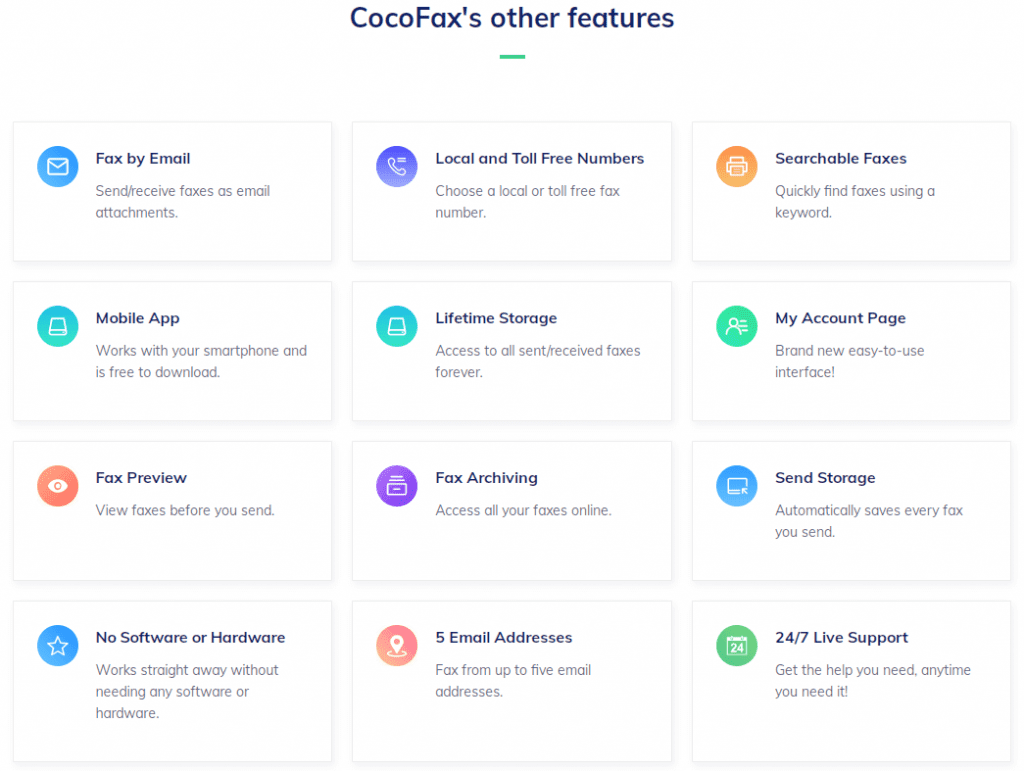This image appears to be a screenshot of a computer interface featuring a service called "Coco Faxes" and its various features, all presented against a white background with black text. At the top, the title "Coco Faxes Other Features" is displayed prominently, underlined by a thin green line. Below, the interface is organized into a grid composed of twelve smaller rectangles arranged in a 3x4 formation, forming a slightly rectangular box. Each rectangle represents a different feature of the service, indicated by both text and an icon.

In the top left corner, a blue circle with an envelope symbol signifies the "Fax by Email" feature, which allows users to send and receive faxes as email attachments. Next to it, a purple circle with a telephone icon denotes the "Local and Toll-Free Numbers" option, which lets users choose a local or toll-free fax number. The third feature, indicated by another icon, is "Searchable Faxes," found in the same row.

The second row includes the following features:
- "Mobile App," which suggests the availability of a mobile application
- "Lifetime Storage," indicating permanent storage capabilities for faxes
- "My Account Page," likely referring to a user account management section

In the third row, the features listed are:
- "Fax Preview," which probably provides a way to preview faxes before sending or receiving
- "Fax Archiving," which offers options to archive faxes systematically
- "Send Storage," hinting at capabilities for storing sent faxes

The bottom row features three more functionalities:
- "No Software or Hardware Requirement," suggesting the service operates without the need for additional software or hardware installations
- "Five Email Addresses," indicating that users can use up to five email addresses for faxing purposes
- "24/7 Live Support," which promises round-the-clock live customer support

Overall, this screenshot serves as a comprehensive overview of the features offered by Coco Faxes, each represented by a distinct icon and brief description.